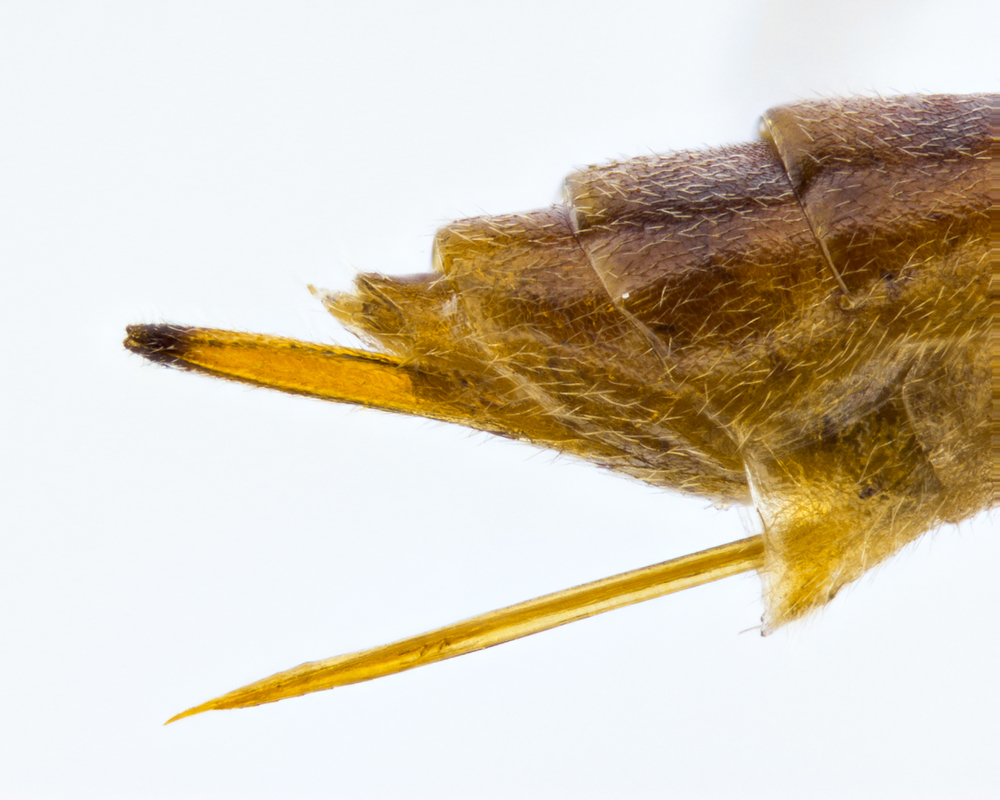The image is a close-up of a mysterious, amber-brown translucent shell or layer, potentially belonging to an insect or small animal. This shell features hair-like structures and multiple overlapping layers, creating an intricate and abstract pattern. The top part of the shell shows gradients of dark brown and black, transitioning into yellow and gold hues, adding to its complexity. There are also two thin, stick-like objects protruding from beneath the layers, which are in a similar golden color. The intricate, almost concentric wrapping of the layers and hairs creates a mesmerizing, yet ambiguous, visual. All of this is set against a stark white background, which adds to the surreal and detailed nature of the image.